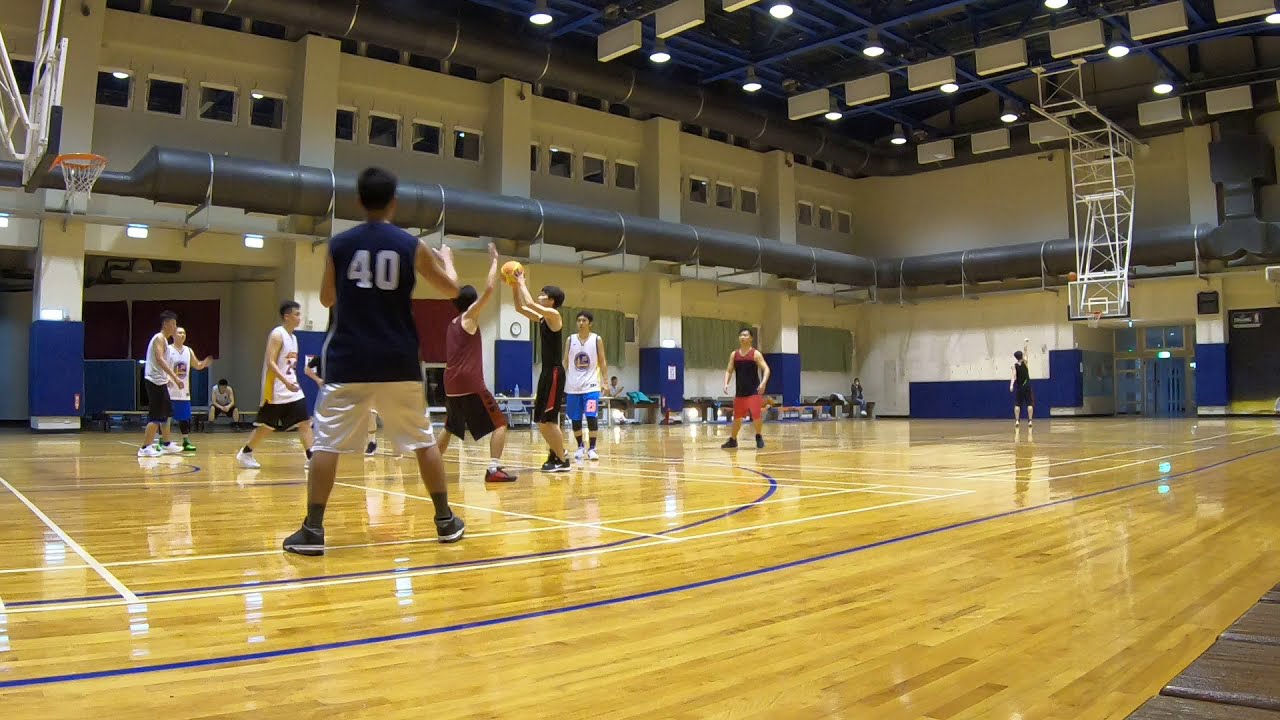The image showcases a horizontally aligned rectangular indoor basketball gym. The court features a light wood color with a highly reflective surface, adorned with blue and white lines. Suspended from the ceiling are supports for the basketball hoops on either side, characterized by white structures and clear acrylic backboards with white rims and orange nets. At each end of the court, basketball goals are visible, one in the upper left and the other in the upper right of the image.

In the center of the gym, several players are engaged in a game. One player, wearing a sleeveless blue jersey with the number 40 printed in white and matching white gym shorts, stands closest to the viewer, preparing to throw the basketball while another player attempts to block him. Among other players, some wear white jerseys with black shorts, while others are adorned in black.

The gym's walls are white, accented with blue padding at the bottom, and a thick gray tube runs through the center of the room. The ceiling is equipped with numerous spotlights and an upper level featuring small square windows, contributing to the brightly lit environment. The entire setting combines standard athletic features with distinct architectural elements, creating an energetic and competitive atmosphere.